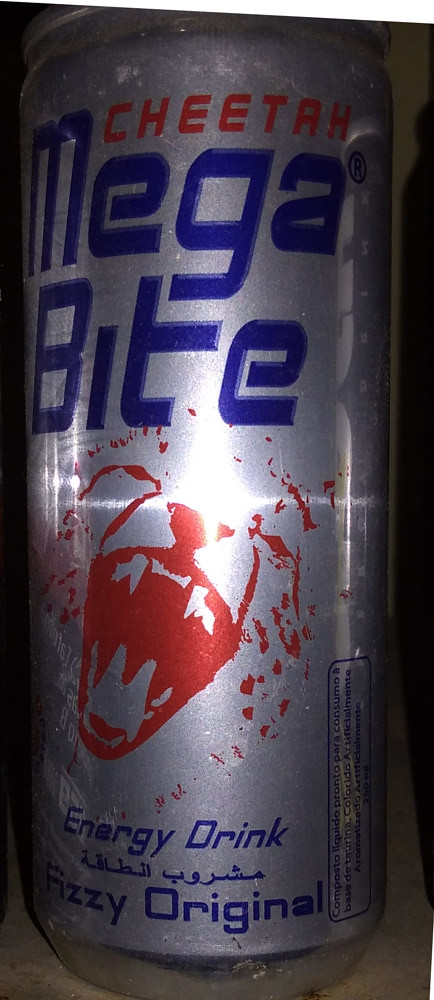This image features a close-up view of an energy drink can. The can is made of silver aluminum and prominently displays a vibrant design. At the top, the word "Cheetah" is written in bold red letters. Below that, "MEGA" is set in large, blue, capital letters, followed by "BITE" in the same style, forming the word "MEGABYTE."

Scattered across the can are small red specks, adding a dynamic touch to the design. Toward the middle of the can, there appears to be an abstract graphic that could be interpreted as a mouth with teeth outlined in red, which ties into the "MEGABYTE" theme. 

Towards the bottom of the can, the phrases "ENERGY DRINK" and "FIZZY ORIGINAL" are printed in blue letters. Additionally, there's some text in a different language, likely Spanish, which presumably provides more details or ingredients of the beverage. This detailed label takes up the entire visible surface in the image, offering a comprehensive look at the product.